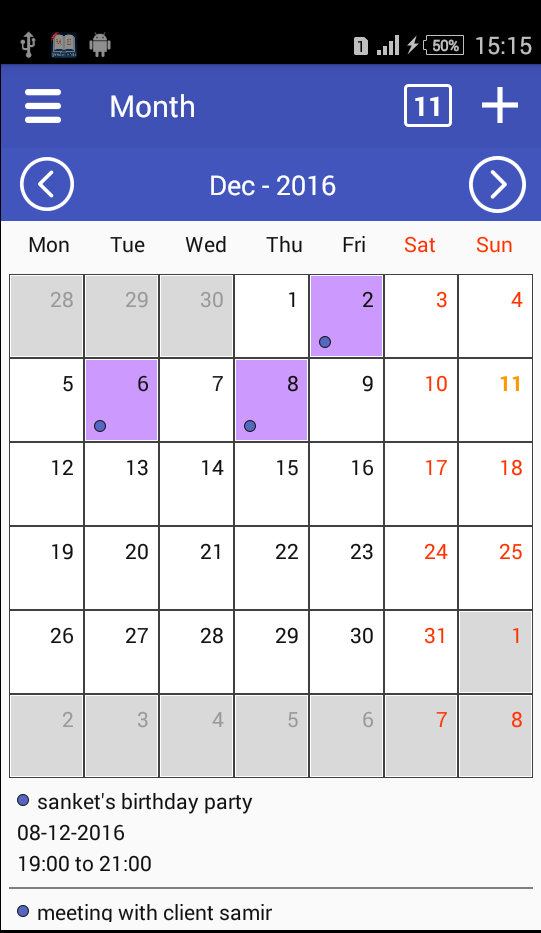This image is a detailed screenshot of a calendar application on a tablet or smartphone, displaying the interface and various notifications. The top section features a black strip with several icons: a USB connection icon, an open book symbol with the letters "U" and "E" in red on each page, a small android character, and a SIM card icon with a number 1 on it. The device shows a full 4-bar cell signal, a battery level at 50%, and the time noted as 3:15 PM.

Below this, the screen transitions into a light purple to purple-blue gradient background. On the upper left, three white horizontal stripes hint at a drop-down menu. The word "month" appears prominently, and to the far right, a square with the number "11" and a plus sign is visible. The current month is December 2016, navigable by arrows on either side.

The calendar spans Monday to Sunday, with weekends (Saturday and Sunday) marked in red. Specific dates, the 6th and 8th of December, are highlighted in lilac, each featuring a small blue dot in the bottom left corner. A caption at the bottom identifies these events: the blue dot on December 8th corresponds to "Sanket's birthday party" from 7:00 PM to 9:00 PM, and another blue dot indicates a "meeting with client Samir." The purpose of the third blue dot remains unspecified.